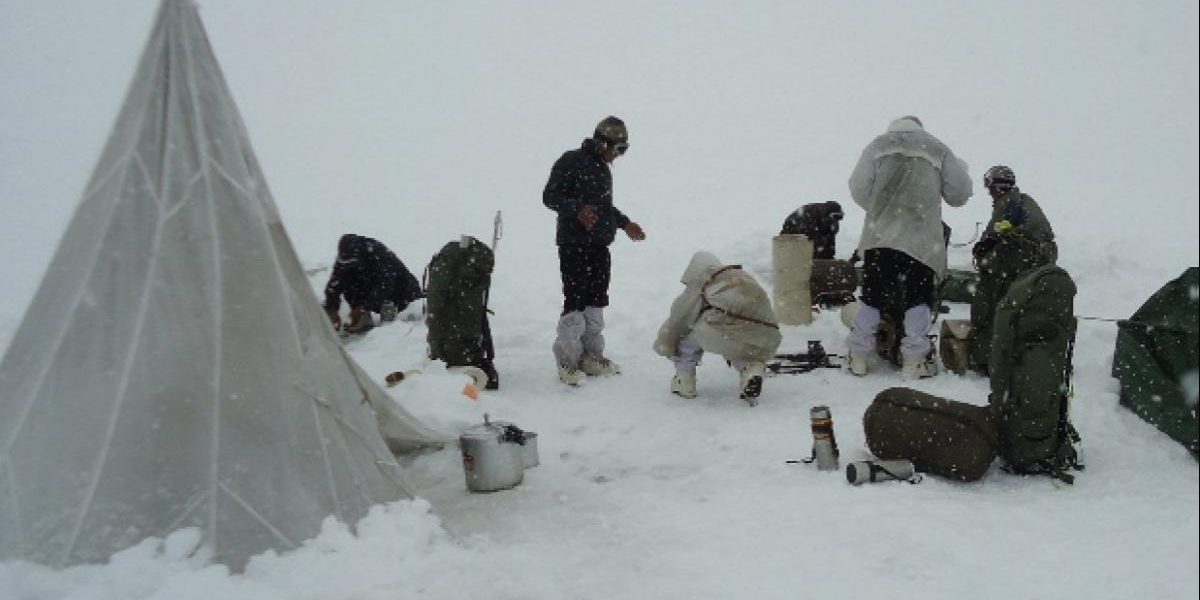In the image, a group of seven people is gathered outdoors in a heavy, thick snow-covered landscape, with the snowfall still ongoing. The background is solid white, indicating an immense snowfall. A gray, teepee-shaped tent stands off to the left-hand side, rounded at the bottom and tapering to a point at the top. In front of the tent, a pot or similar cooking utensil is visible, suggesting they may have been cooking or preparing food. The ground is littered with various camping equipment including large backpacks, thermoses, and other utensils, hinting that they camped there overnight and are in the process of packing up.

The individuals, comprised likely of men, are wearing thick snow boots, heavy jackets, snow pants, goggles, and hats, indicating the cold and extreme weather conditions. One person is kneeling in the snow, seemingly occupied with a task, another appears to be tying their shoe, and three others are sitting in a small group. The rest are either standing or squatting around, bundled up in variously colored winter clothing—some in black coats and pants, others in white, and one in olive green. The heavy snowfall and the detailed gear of the campers provide a vivid image of the harsh, wintry environment they are navigating.